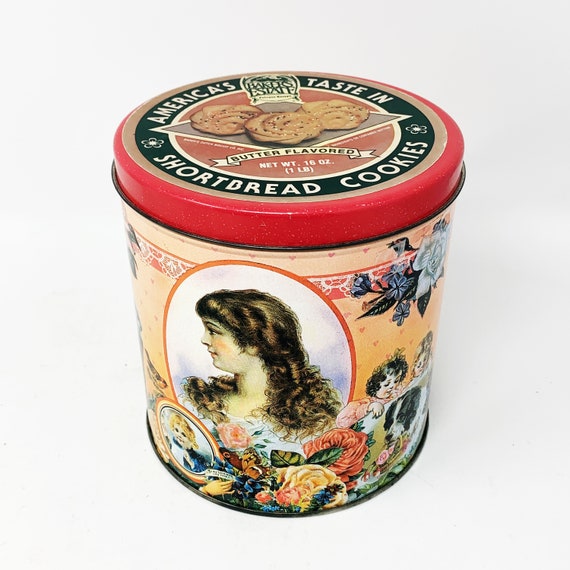The object is a very old, vintage-style tin canister of shortbread cookies, reminiscent of the 1900s, with possible Victorian influences. The lid is adorned with a red brim and features a circular label reading, "America's Taste in Shortbread Cookies, Butter Flavored," encircling an image of three shortbread cookies. The tin itself is primarily a buttery yellow or peach color and is intricately decorated with vibrant, colorful flowers. One of the main visual elements on the side of the tin is a portrait of a young girl with long, wavy, dark brown hair and blushed cheeks, wearing a dress and looking sideways. Below her portrait is a smaller image of a blonde girl in an apron. Additional illustrations around the tin include various children and a brown and white dog, contributing to the overall nostalgic and charming aesthetic. The weight of the contents is marked as one pound, 16 ounces on the lid.